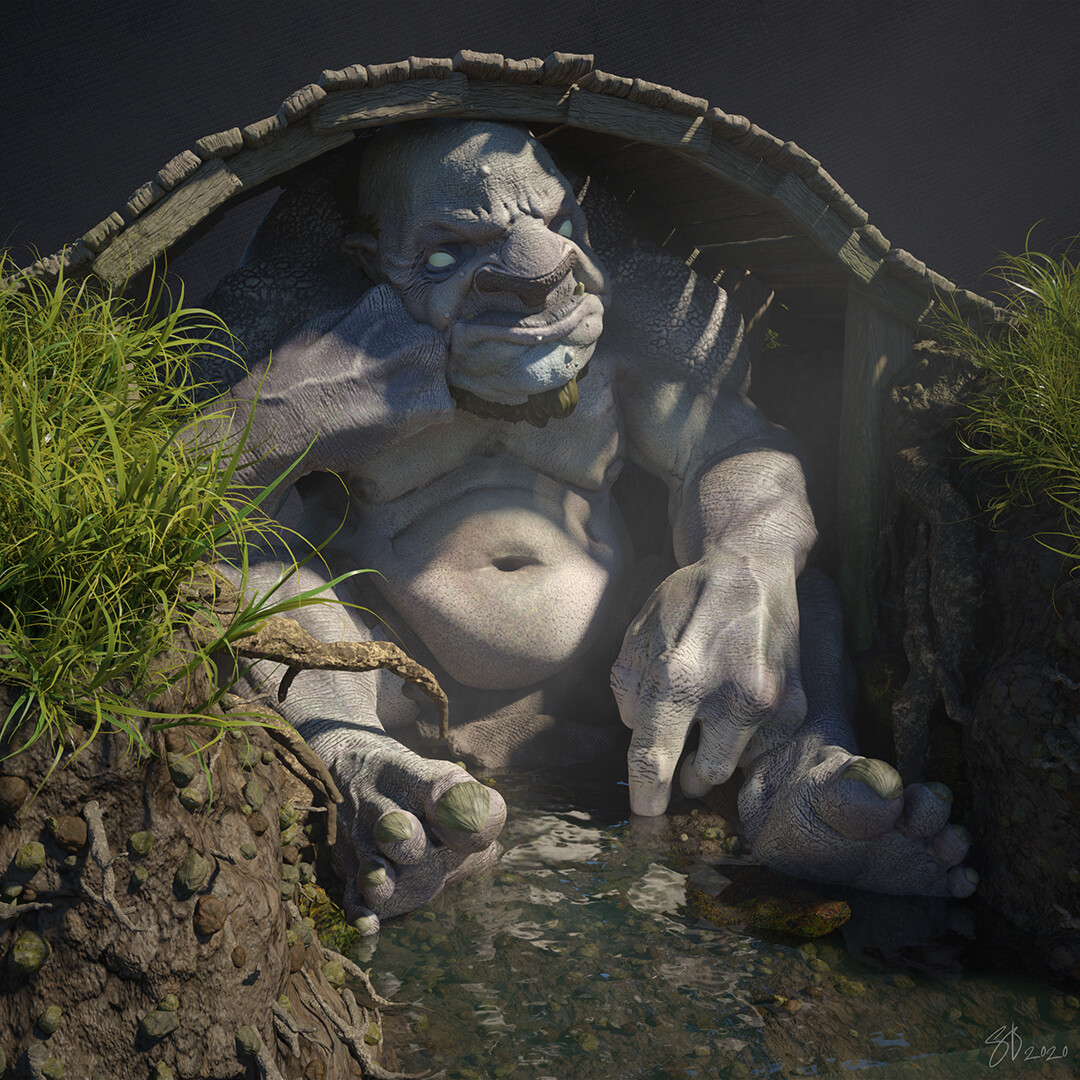This outdoor photograph, almost square in shape, captures a detailed and vivid scene featuring a garden fountain sculpture. At the bottom center of the image, the water gently flows among scattered rocks, reflecting the daylight. At the heart of this setting, a gray, concrete statue of a squat, gargoyle-like demon sits beneath an arching, bridge-like structure crafted to resemble wooden planks but made of lighter gray concrete. The figure, with a large, round head adorned with pointed ears and white, uncolored eyes, exhibits a distorted, snarling face with a flattened nose and horselike mouth. Its robust body displays a prominent pot belly, covered partially by a concrete cloth between its legs, and it has massive feet submerged in the water. One finger of its enormous hands points towards the stream, completing the haunting and captivating presence of the statue that appears to guard this small, mystical water feature. The backdrop fades into dark emptiness, drawing all focus to the intricate details of the fountain sculpture and its immediate surroundings, which include patches of dirt and grass with visible roots.